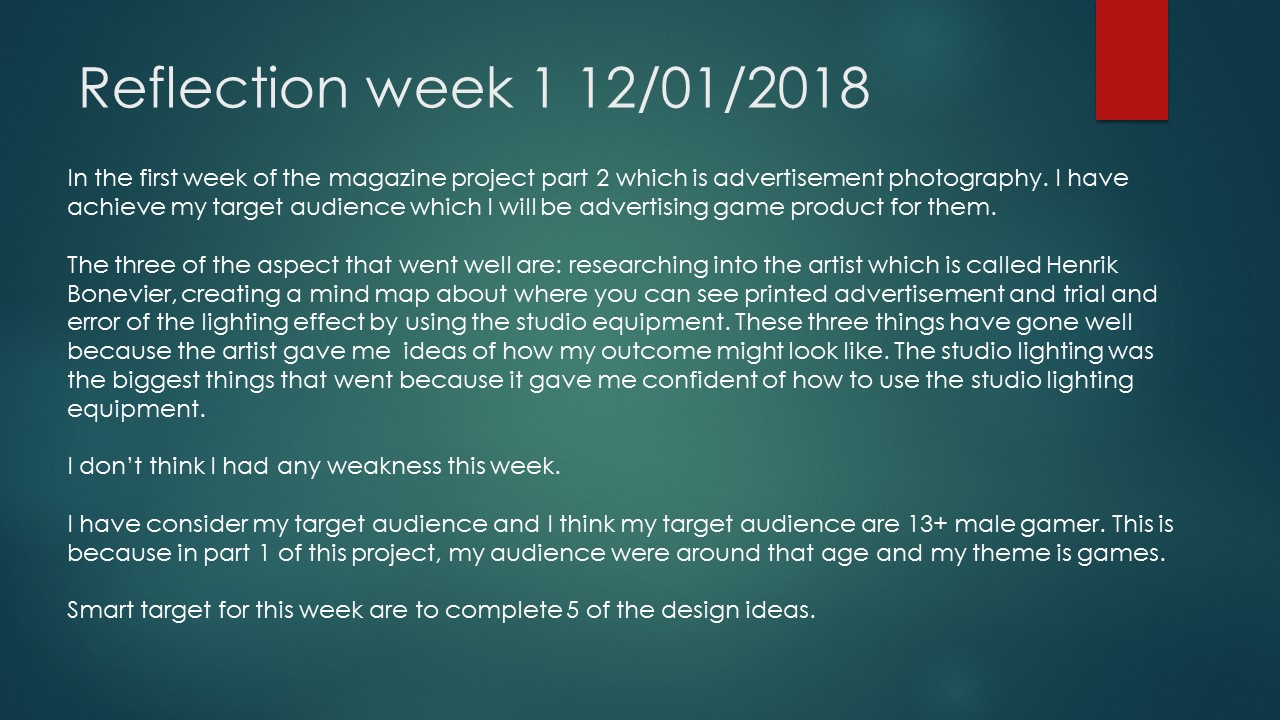The image depicts a slide from a presentation card with a horizontally oriented layout. The background features a gradient green color, transitioning from a lighter shade in the middle to a darker one at the edges. The top left corner contains the title "Reflection Week 1, 12-01-2018" written in white text. Below this title, the body text describes achievements and reflections from the first week of the Magazine Project Part 2, focused on Advertisement Photography. Specifically, the presenter mentions having successfully targeted their audience, intending to advertise a game product to them.

The slide details that three aspects that went well include researching the artist Henrik Bonnevier, creating a mind map for printed advertisements, and experimenting with studio lighting equipment. Additional comments note that insights from Henrik Bonnevier influenced the project outcomes and that mastering studio lighting boosted the presenter's confidence. Also mentioned is the consideration of a target audience of male gamers aged 13 and above. The card concludes with a "smart target" goal to complete five design ideas within the week. Notably, a small red rectangle is situated in the upper right corner, vertically oriented and around an inch in length.